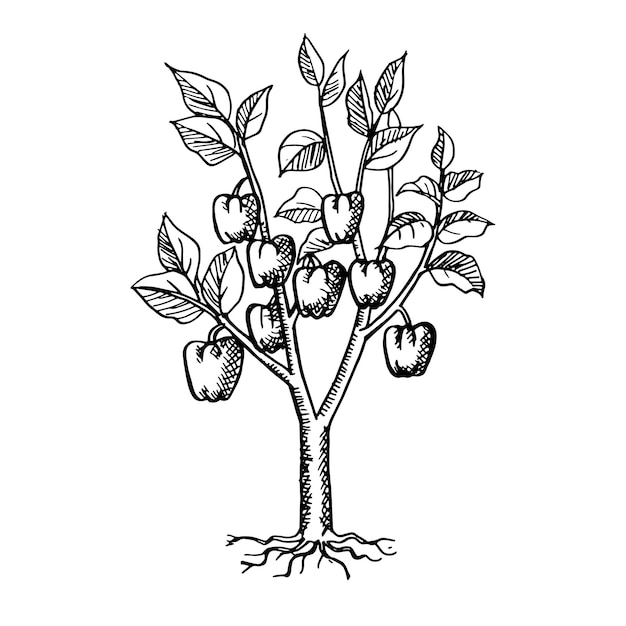This black and white line drawing depicts a plant that resembles either a pepper plant or a small apple tree. The illustration is void of any background elements, focusing solely on the plant itself, with roots exposed at the bottom. The roots are detailed, branching out to the left and right. The main stalk rises and splits into two primary branches, which then further divide into smaller branches. Hatch marks are used on the tree trunk to add texture and detail. The branches are adorned with leaves and feature a total of eight hanging fruits, which look like bell peppers but might also be interpreted as apples. The simplicity of the black and white contrast emphasizes the plant’s structure and form, lacking any additional color or backdrop.